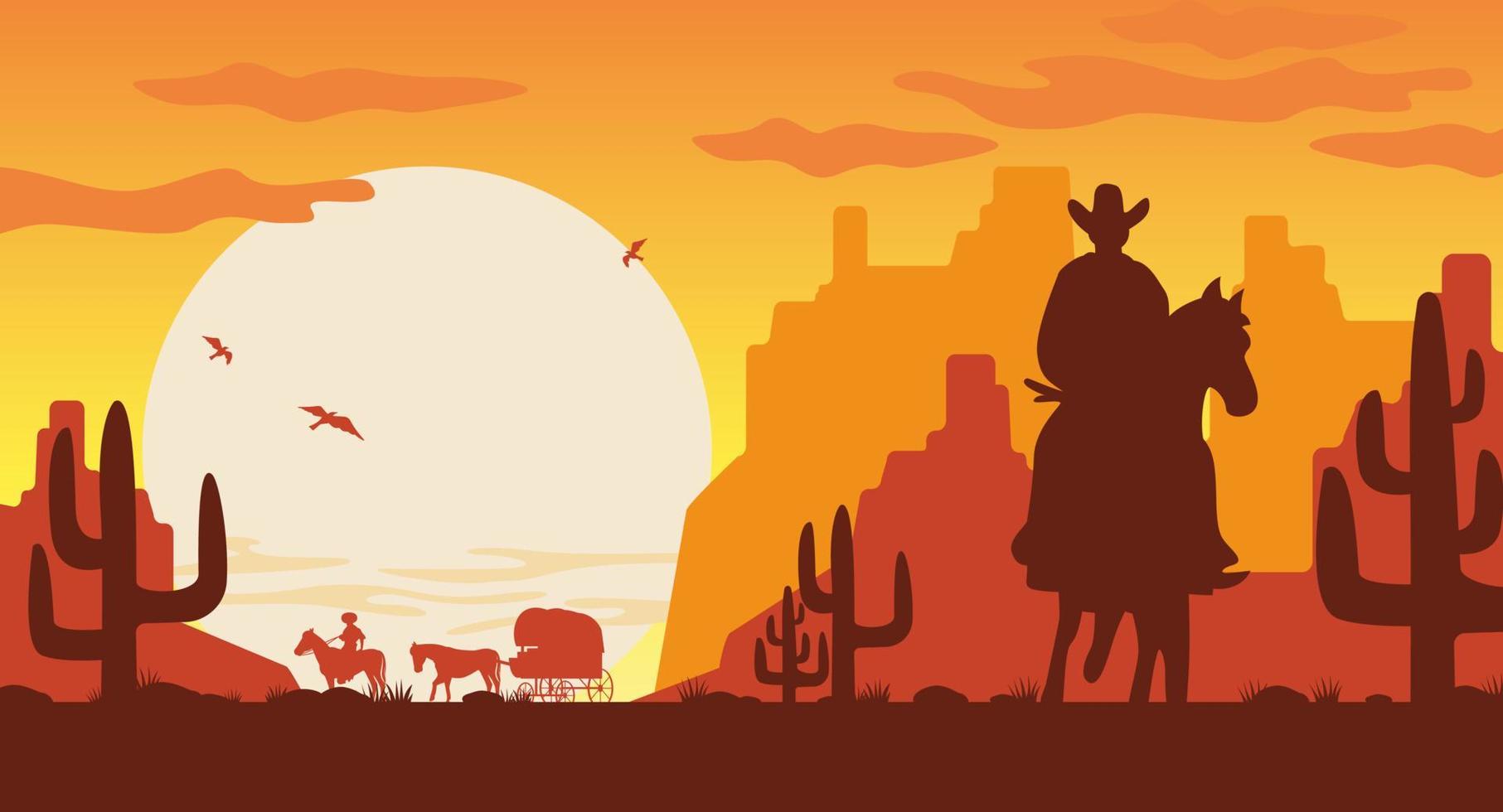This is a large rectangular poster with a western theme, showcasing a vivid desert landscape. Dominated by an orange background, the scene is bathed in hues of red and yellow, evoking the ambience of the Wild West. A silhouette of a cowboy riding a horse commands the foreground, to the right of which stands a cactus with three outstretched arms. Additional cacti dot the terrain, fading into the distance against the silhouettes of towering plateaus and rugged rock formations reminiscent of those found in Utah or Arizona.

In the middle ground, another cowboy on horseback is seen, trailing a second horse that tows a vintage 1800s-style carriage. This layered composition features darker browns in the foreground, reddish-browns in the midground, and lighter oranges as the scene extends back. The sky is animated with orange-painted clouds, and three birds soar gracefully above.

A prominent feature is the large, circular sun occupying the upper half of the poster, casting its glow over the entire scene. The sky transitions from a light yellow near the horizon to vibrant oranges, giving the impression of dawn breaking over the serene yet rugged landscape. The detailed silhouettes, from the cowboys to the flora and fauna, enrich the portrayal of this timeless western vignette.